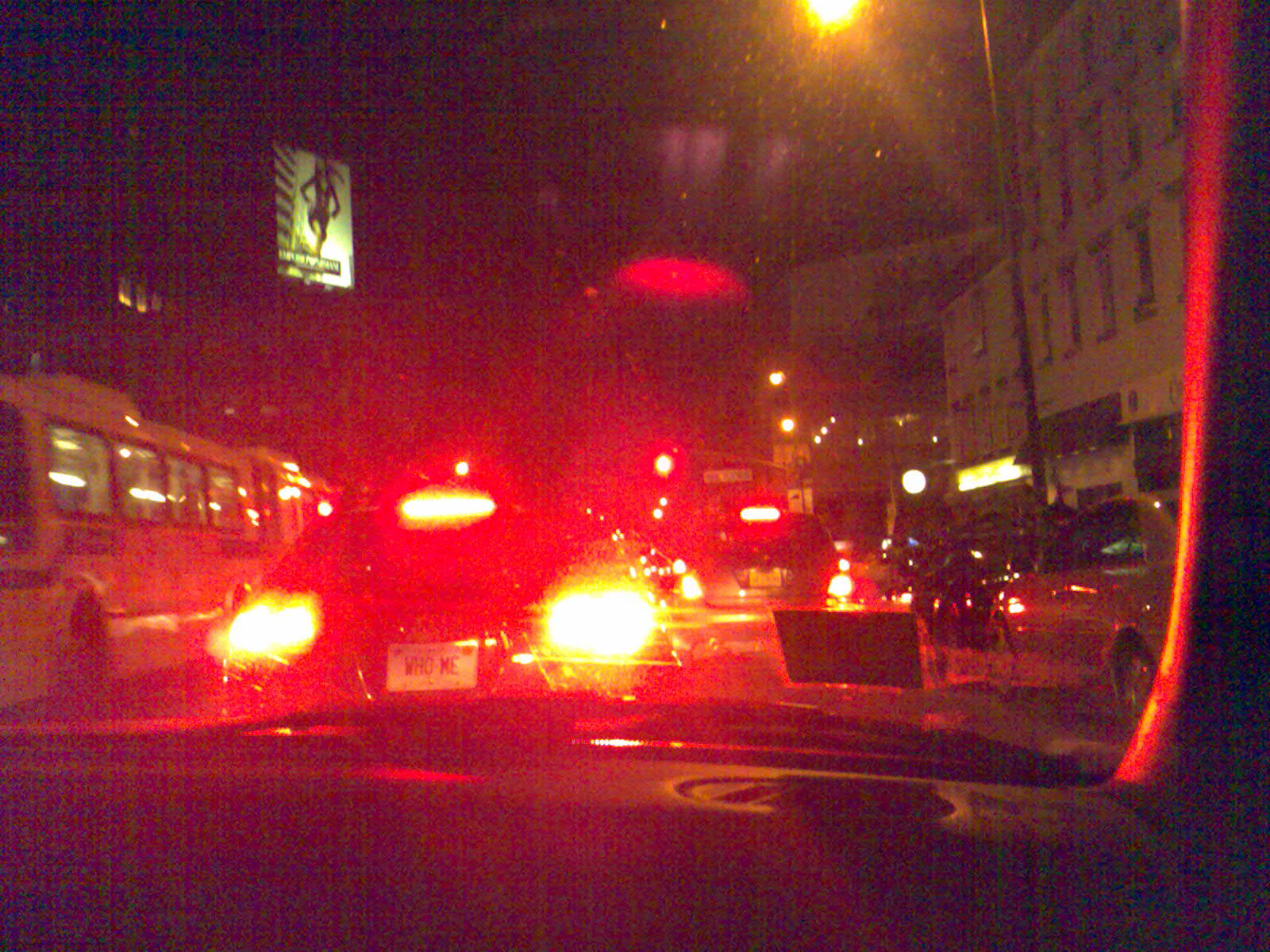This nighttime photograph, taken from inside a car through its windshield, captures a city street alive with activity. The dashboard and interior of the car frame the image, adding context. Directly ahead, a car with bright brake lights casts a red glow over the scene, emphasizing its white license plate that reads "WHO ME." The street is bustling with traffic in both directions, lined with tall buildings on either side. Parked cars are visible, particularly on the right, and a large, white bus occupies the bottom left corner of the frame, recognizable by its numerous windows. Further back, a prominent billboard in the top left corner displays an image of a person dancing or exercising. The illuminated streets feature several streetlights, glowing red from traffic signals, indicating that all vehicles, including the one the photo was taken from, are stopped. Despite the darkness, light poles and some building lights cast a subdued illumination, adding to the atmosphere of the nighttime urban landscape.